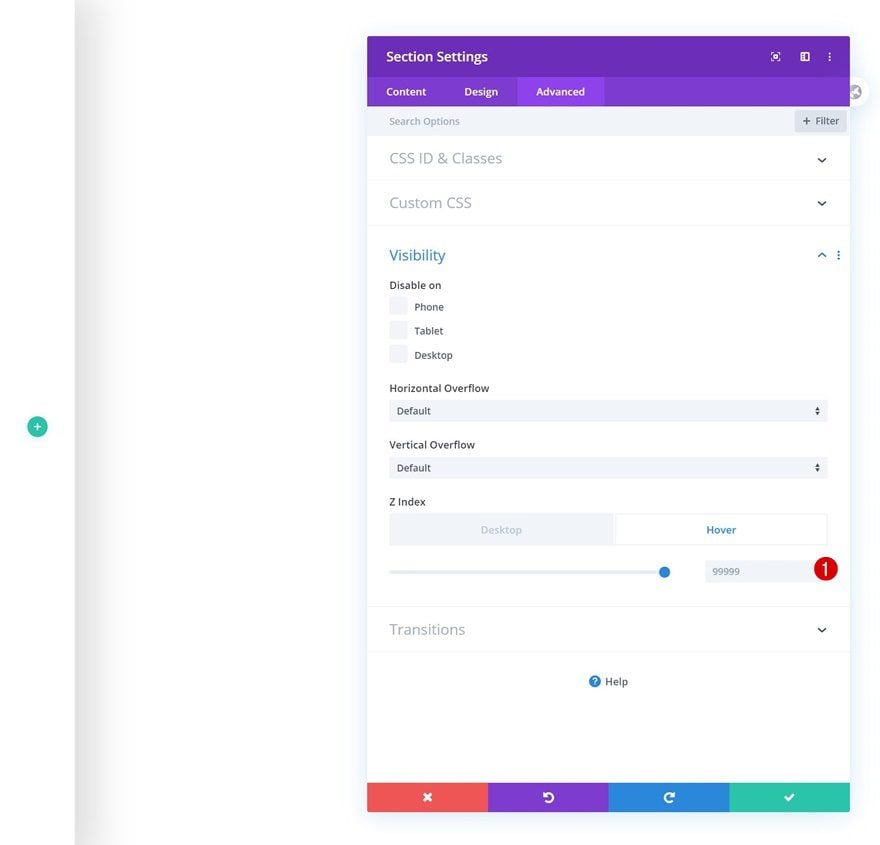At the top of the image, there is a purple rectangular section labeled "Section Settings," with subcategories titled "Content," "Design," and "Advanced." Directly below this, there is a large, empty search bar with a filter option to its right. Below the search bar, bold, uppercase text reads "CSS ID AND CLASSES."

Approximately two inches down, there is a section labeled "Custom CSS." Several inches further down, the word "Visibility" appears in blue. Below the visibility section, there is a "Disable On" feature with options to disable on "Phone," "Tablet," and "Desktop."

Next, there are sections for "Horizontal Overflow" and "Vertical Overflow," both defaulting to unselected options. Following this, there is a section for "Z-Index" with the word "Desktop" underneath. Adjacent to this, a long gray line features a blue circle towards its right end.

Below this, there is an empty rectangular area that contains a sequence of five number nines. Finally, at the very bottom, there is a section labeled "Transitions," followed by four color options: coral pink, purple, blue, and green.